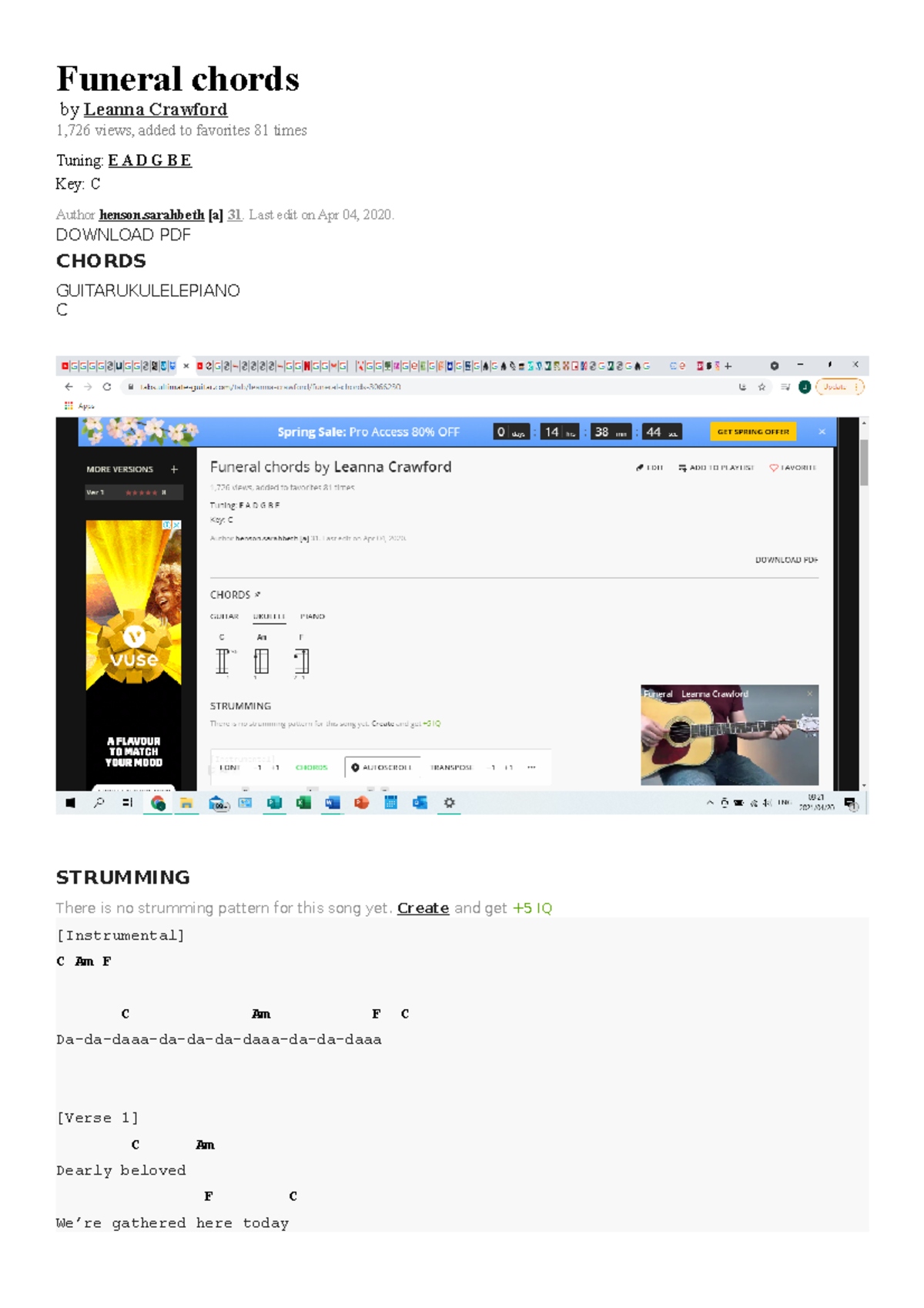Here's a cleaned-up and detailed caption for the image:

---

The image appears to be a screenshot from a web page dedicated to guitar chords for a song titled "Funeral Chords," authored by Lena Crawford. 

In the upper left-hand corner, the title "Funeral Chords" is prominently displayed with smaller black text underneath stating "by Lena Crawford." Below this, in light gray font, it reads "1726 views, added to favorites 81 times." Further down, it indicates the standard guitar tuning "EADGBE," with the key noted as "C." The author's name "Sarah Beth" is noted in smaller text, with the additional detail "last edited on April 4th, 2020" in gray beside it.

The page features several key elements:
- A downloadable PDF link in large black text.
- Bold "Chords" heading, denoting the section for different chords for guitar, ukulele, and piano.
- A visual section with a screenshot, showing a skinny gray bar at the top cluttered with open page icons.
- Below this, a blue bar with a floral motif on the left and right sides, accompanied by the text "Spring Sale Pro Access 80% Off" and a countdown timer indicating "14 hours 38 minutes 44 seconds." There is a yellow box with the prompt "Get Spring Offer" to the right of the timer.

On the left, there is a vertical black box featuring a yellow circle labeled "Fuse." Inside this yellow circle, a white smaller circle displays a yellow "V." Adjacent to this, a woman is seen, and below in white text, it says "A flavor to match your mood."

The main body of the web page, against a white background, centrally highlights "Funeral Chords by Lena Crawford." Information about various chords and their finger positions on a guitar is provided. An image at the bottom right captures a person wearing jeans and a burgundy short-sleeved shirt, strumming a guitar on their lap.

Beneath this main section is a skinny gray bar lined with icons. Another text box follows, titled "Strumming," mentioning that "There is no strumming pattern for this song yet. Create and get +5 IQ." Lastly, a gray box with black text gives detailed information on the chords and strumming patterns.

---

This detailed caption encapsulates the key features and structure of the web page, providing clear descriptions of both text and visual elements.